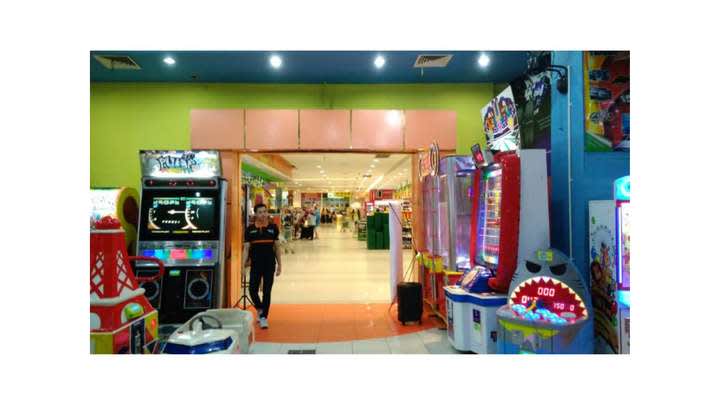The photograph showcases a vibrant arcade situated inside a shopping mall. The arcade room features lime green walls and a light blue ceiling with ample lighting. A solitary male worker, identifiable by his black and orange uniform, short black hair, and white sneakers, is seen walking towards the viewer. The arcade is filled with a diverse array of colorful games and attractions, including a claw machine, a rocking fake automobile ride, and a game resembling an angry shark with a screen displaying "000." The array of machines also includes a shooting game to the left and glass-encased vending or coin games on the right. The background of the image shows more visitors and shops, indicating a lively, well-lit shopping mall environment. The overall scene is rich in colors, including black, white, gray, green, blue, red, pink, yellow, orange, and purple, despite the image's pixelated, low-resolution quality.